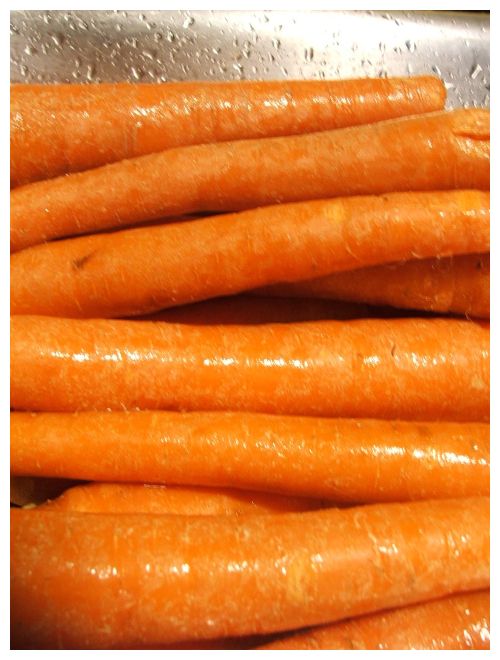This photograph is an extreme close-up of a pile of vibrant, bright orange carrots. The carrots, numbering around nine to twelve, are arranged horizontally in an unidentified metal container, likely stainless steel or aluminum, evident from the glistening water droplets covering both the container's surface and the carrots. The carrots appear freshly washed, their smooth skins reflecting light due to the residual water. The ends of the carrots have been neatly cut off, although they have not been peeled, preserving their natural texture. Subtle imperfections, such as slight bruising on a few carrots, are discernible, adding to the realistic depiction of the freshly cleaned produce, seemingly prepped for cooking or packaging. The photograph's focal lighting enhances the carrots' vibrant color and moist surface, forming a striking contrast with the metal container in the background.